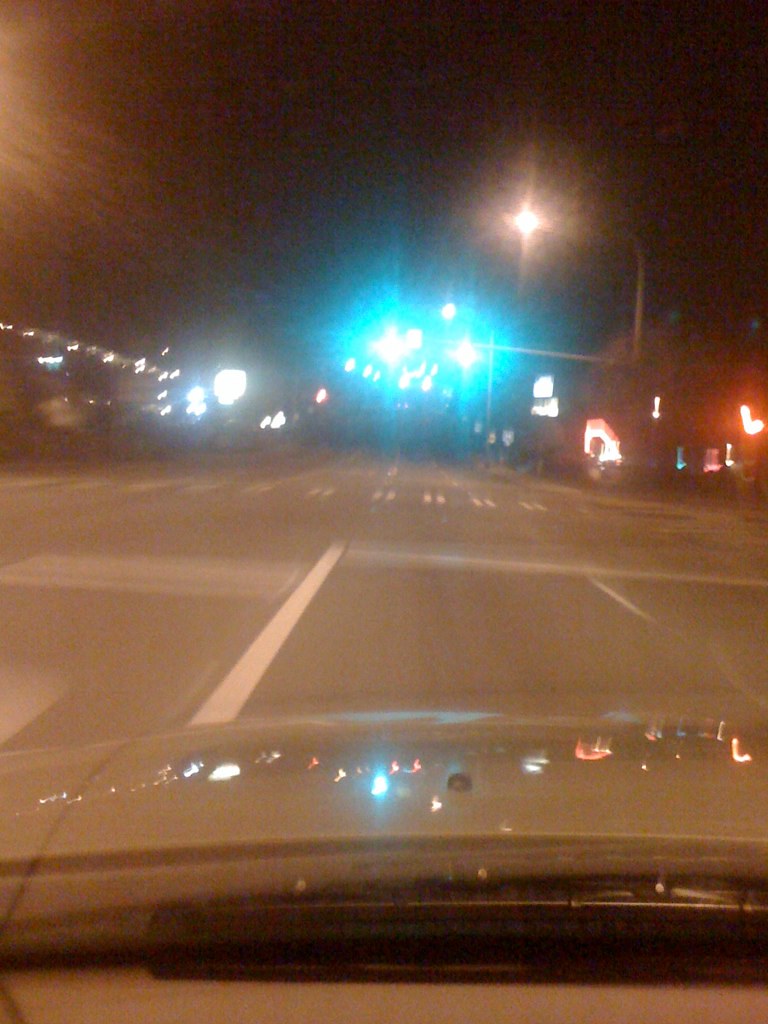The image, taken from inside a vehicle at night, offers a blurry yet atmospheric view from the driver's perspective. The white hood of the car, partially blocked by black windshield wipers, is illuminated by a myriad of colorful lights reflecting off its surface. Ahead, an intersection appears under poorly defined yet colorful light, predominantly with a blue and green hue. The glowing lights suggest the presence of a traffic signal, albeit the specifics are obscured by the darkness and camera limitations. The roadway, seemingly a four-lane street, is devoid of other vehicles, emphasizing the late hour. On either side of the street, the dim outlines of buildings can be seen, their shapes indistinct but adorned with various illuminated signs and lights. Words painted on the asphalt are partially visible but unreadable, and a bright orange crossing signal gleams against the night. Further down, additional streetlights cast an orange glow, enhancing the scene's night-time ambiance.